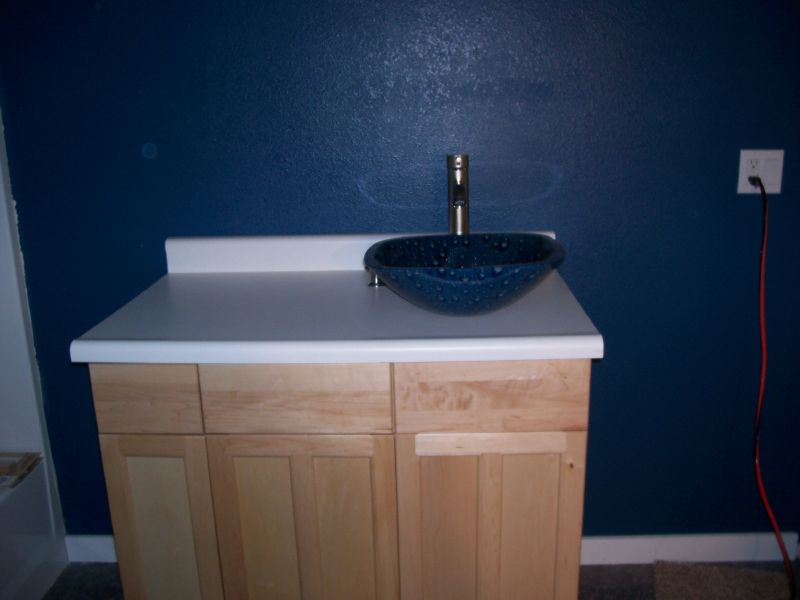The image showcases a modern bathroom with a focus on the sink and its supporting cabinetry. The sink itself is a striking blue ceramic bowl that sits atop the counter, without any recess into the cabinetry, providing a contemporary aesthetic. A chrome faucet with a lever handle, used to control water temperature by lifting and turning side to side, adorns the sink. 

Beneath the sink, a visible pipe extends straight down into the cabinetry below and subsequently into the wall, emphasizing the external nature of the basin. To the right of the sink, mounted on the wall at approximately chest height, is a US-style electrical outlet with two sockets, one on top of the other. The bottom socket is occupied by a plug attached to a cable that features alternating black and red stripes, the destination and purpose of which are not clear. This detailed depiction highlights the modern design and functional elements of the bathroom setup.